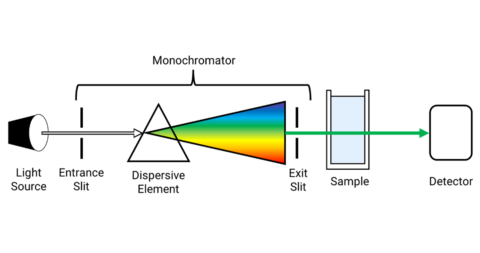The diagram illustrates the operation of a monochromator, presented in a sequential left-to-right arrangement. At the top center of the rectangular image, the word "Monochromator" is prominently displayed in black lettering. The process begins with a "Light Source" depicted as a black tube with a white center located on the left side. This tube directs light into the "Entrance Slit," which is the first of two vertical black bars positioned on either side of a triangle.

Labeled "Dispersive Element," this triangle has its point facing left and its base extending to the right, exhibiting a gradual color transition from dark blue at the top to orange at the bottom, symbolizing the dispersion of light into a spectrum. The apex of the triangle, where the light enters, is followed by a "Rainbow Triangle" that further disperses the light.

A green arrow originates at the base of the triangle, extending through the "Exit Slit"—the second vertical black bar—to a rectangular box labeled "Sample." This box is light blue with a white border, representing a sample container. The green arrow continues from the sample to a square outline labeled "Detector," situated at the far right end of the diagram.

The overall assembly of these components, connected by labeled lines and arrows, provides a clear visualization of how light moves from the source, through the monochromator, is dispersed by the prism, passes through the sample, and is finally detected.